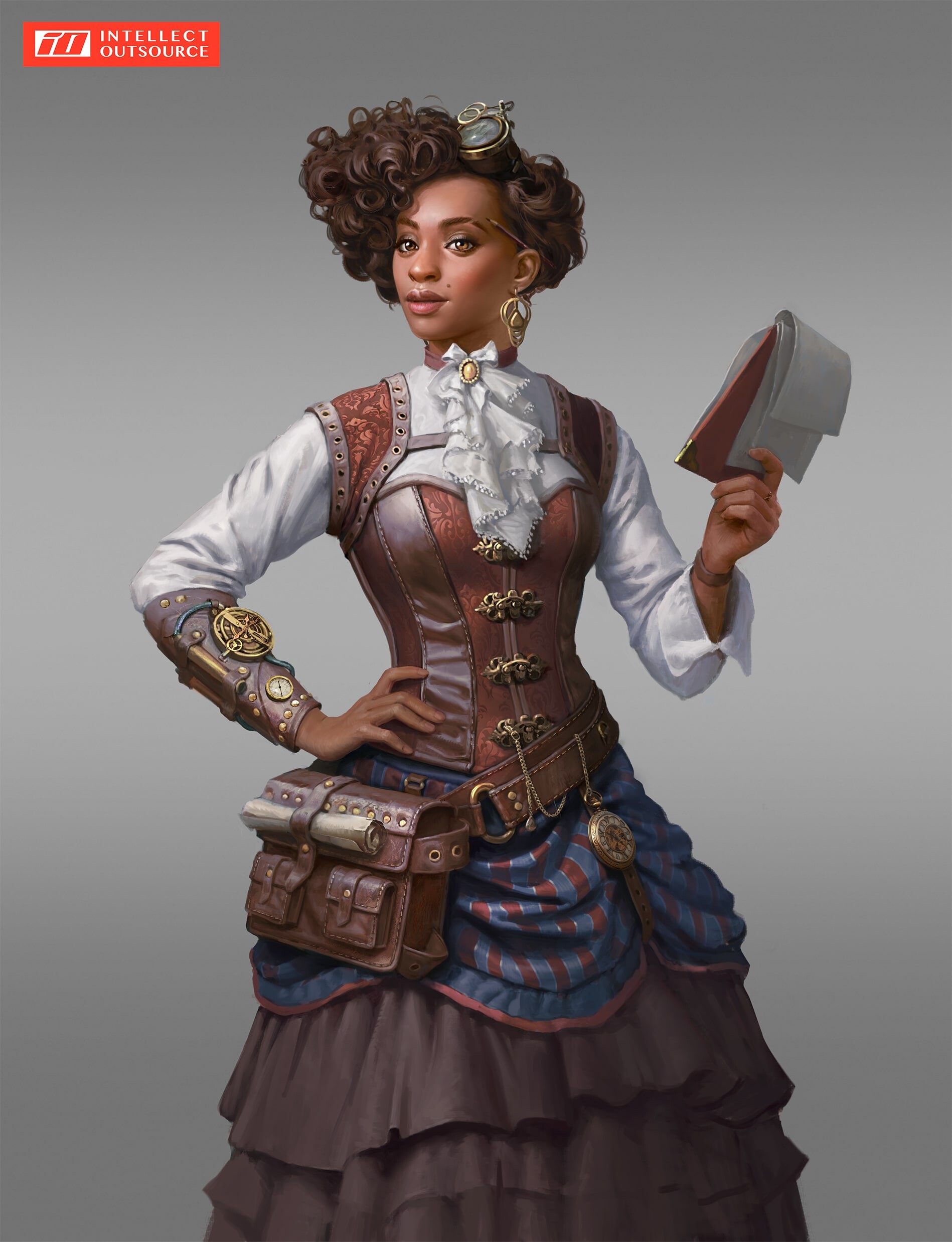The image depicts a highly detailed and realistic CGI-rendered or concept art portrait of a tan-skinned woman, set against a gray background. In the upper left-hand corner, there's a red rectangle logo featuring "IO" in white, alongside the words "Intellect Outsource" in white lettering. The woman is centered in the image, her head stopping short of the top edge, while the bottom edge is obscured by the layered and ruffled hem of her voluminous dress.

Her attire is a blend of steampunk and western styles. She wears curly black hair pinned up with steampunk goggles and a pencil tucked behind her ear. There’s a noticeable earring in her left ear, and her body is slightly turned to her left, offering a view of the left side of her face. Her white blouse is adorned with ruffles at the front, and two pieces of fabric drape over her shoulders, transitioning into a leather corset-like garment beneath, fastened with buckles. Just below, she dons a blue and red ruffled skirt that fades into dark gray or brown at the bottom.

Her right arm bent, hand resting on her hip, reveals a metal band or leather gauntlet on her forearm and a thick-banded watch on her wrist. Her left hand extends outward, clutching a notepad. Around her waist is a brown leather belt, from which hangs a small leather bag brimming with rolled-up papers. A pocket watch dangles from the belt on her left side.

Overall, the scene is bathed in bright, clear lighting, highlighting the intricate details of the woman's steampunk-inspired ensemble and accessories.